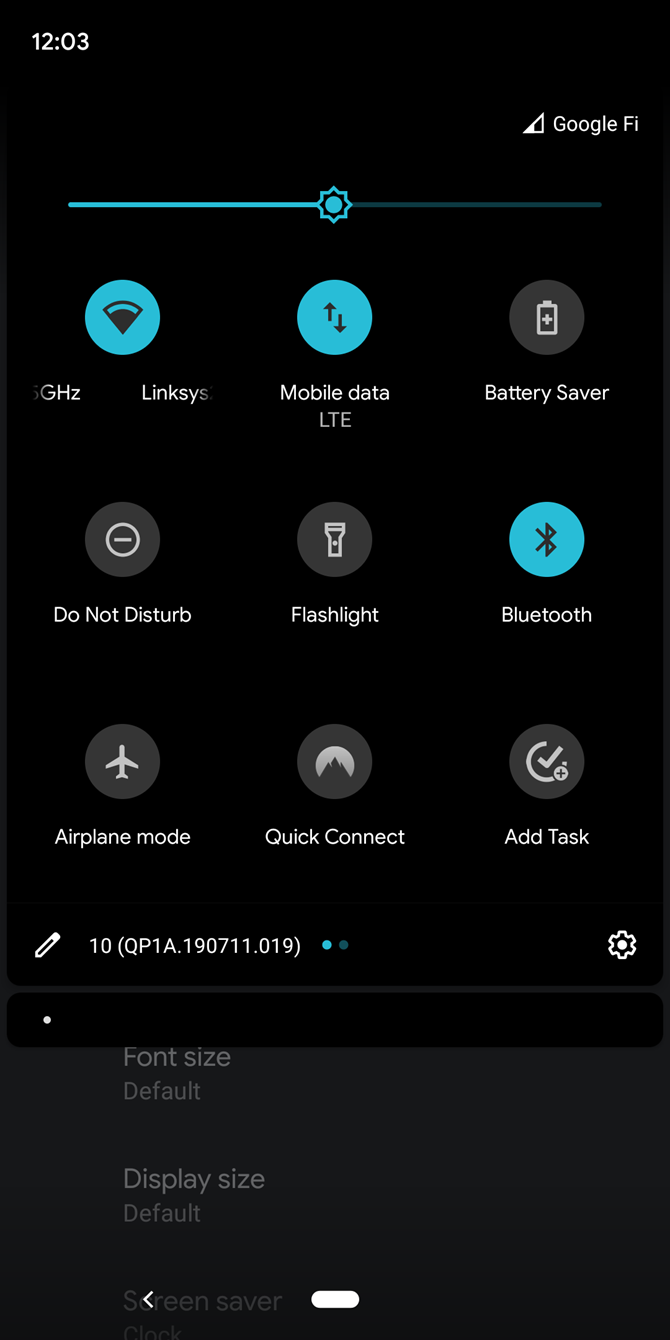Here is a cleaned-up version of the descriptive caption, providing detailed information about the screenshot:

---

The image is a screenshot of a smartphone's notification and settings panel. The user has swiped down from the top of the homepage, revealing various quick settings options. The Wi-Fi is activated, indicated by a highlighted icon. Mobile data is also enabled, showing LTE connectivity. The Battery Saver and Do Not Disturb options are present but turned off. The Flashlight is also off, while the Bluetooth is on, marked by a blue icon. Additionally, Airplane Mode and Quick Connect are both off. 

In the top right corner, there is a settings gear icon. Notably, there is a version number displayed, "10 (QP1A.190711.019)," though its significance is unclear—possibly an OS version or network identifier.

Further down, the screen shows settings options including Font Size (set to default), Display Size (also at default), and the Screensaver setting, which is partially cut off in the image. The background of the screen is black, with white text and icons. Selected options are highlighted in blue for clear visual indication.

---